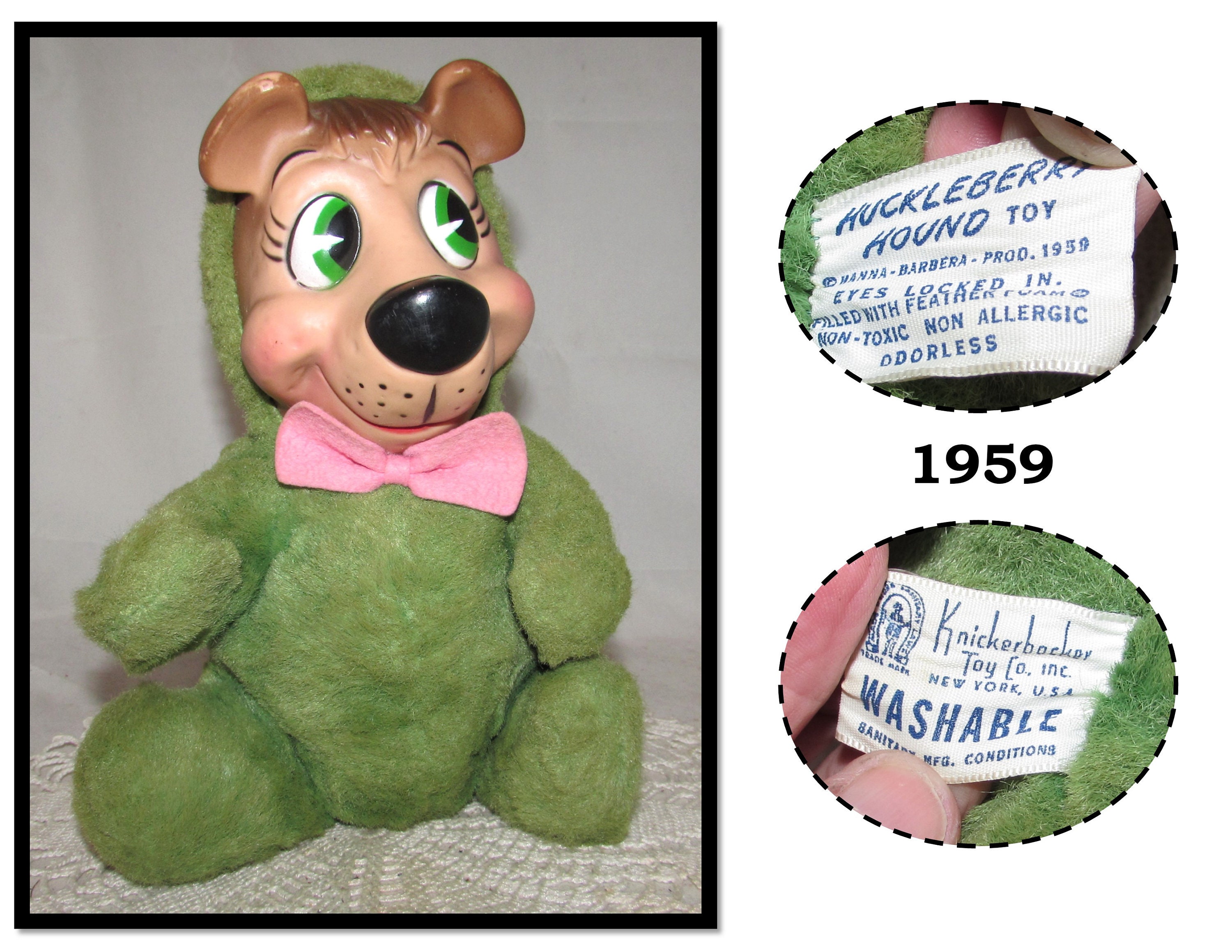The image is a detailed photograph featuring an old stuffed teddy bear. The bear has a distinctive design with a mossy green, soft-textured body, and a hard plastic face. Its facial features include green eyes, a big black nose, painted whiskers, eyelashes, and rosy cheeks, topped with brown hair and plastic ears. The bear is adorned with a pink bow tie around its neck. 

Positioned next to the bear are two oval images displaying important information about the toy. The first oval tag identifies it as a "Huckleberry Hound Toy," produced in 1959, emphasizing that the eyes are securely locked in, and the bear is filled with feather foam. The tags highlight that the toy is non-toxic, non-allergenic, and odorless, assuring its safety for children. 

The second oval tag reveals the manufacturer, the Knickerbocker Toy Co., Incorporated, based in New York, USA, and adds that the toy is washable and produced under sanitary conditions, although part of this text is obscured by someone's fingers.